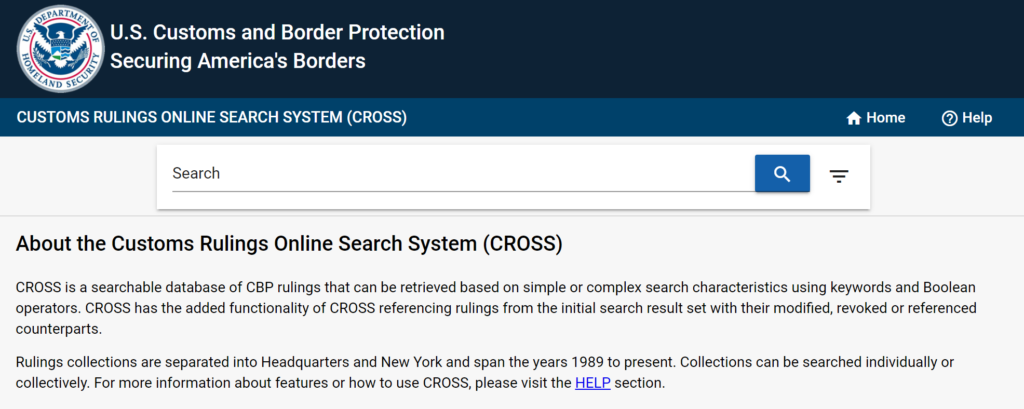This is a detailed screenshot taken from a section of the U.S. Customs and Border Protection website. The top of the image features a very dark blue banner displaying the U.S. Department of Homeland Security logo on the upper left. The logo showcases an eagle with a shield positioned in front of it, atop blue mountains set against a white background. To the right of the logo, the banner reads "U.S. Customs and Border Protection Securing America's Borders."

Beneath this, there's a lighter blue banner with white text that states "Customs Rulings Online Search System" or "CROSS," flanked by home and help buttons. Directly below these buttons is a search field. The description under the search field reads:

"About the Customs Ruling Online Search System, CROSS. CROSS is a searchable database of CBP rulings that can be retrieved based on simple or complex search characteristics using keywords and boolean operators. CROSS has the added functionality of cross-referencing rulings from the initial search results set with their modified, revoked, or referenced counterparts. Rulings collections are separated into headquarters in New York and span the years 1989 to present. Collections can be searched individually or collectively. For more information about features or how to use CROSS, please visit the help section."

The word "help" in the help section is a hyperlink, highlighted in blue and underlined.